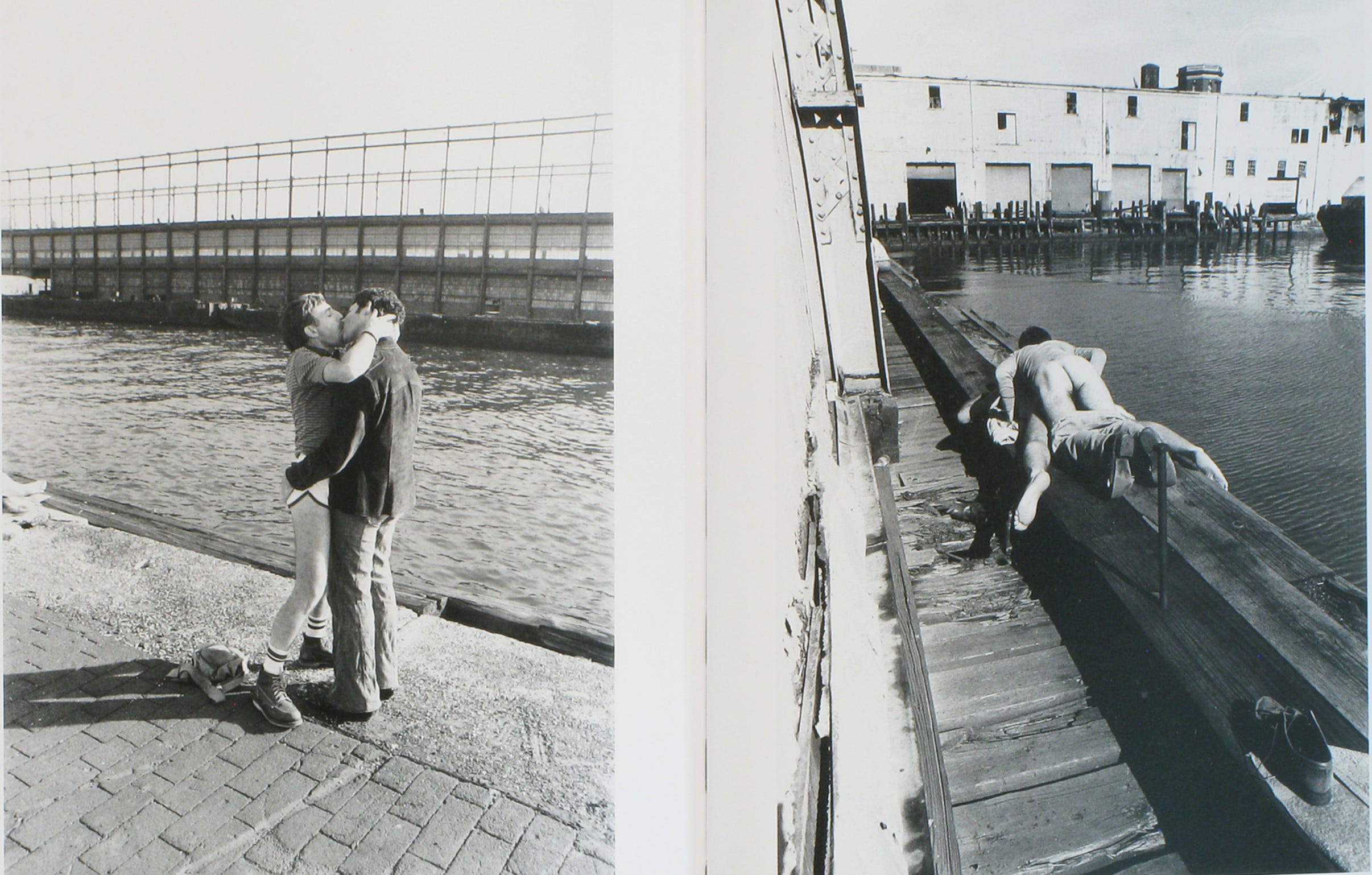This horizontally rectangular black and white image features two vertically rectangular photographs side by side. The left photograph captures a tender moment between two men in front of a body of water, possibly near a dock. One man is dressed in white short shorts with a black hem, white socks with black rings, boots, and a dark striped shirt, evoking a retro 80s style. His partner wears a long-sleeved dark-colored shirt and medium-colored pants. They are standing on a paved walkway, and a bridge can be seen in the background.

The right photograph appears more explicit and portrays two men in an intimate act. One man is laying on top of the other, with his pants down to his knees, exposing his bare buttocks. Only the leg and shoes of the man underneath are visible. This scene takes place next to a wooden railing by the water, and an old building is visible in the background. While the faces of the men are obscured, the rawness of the moment is vividly captured.